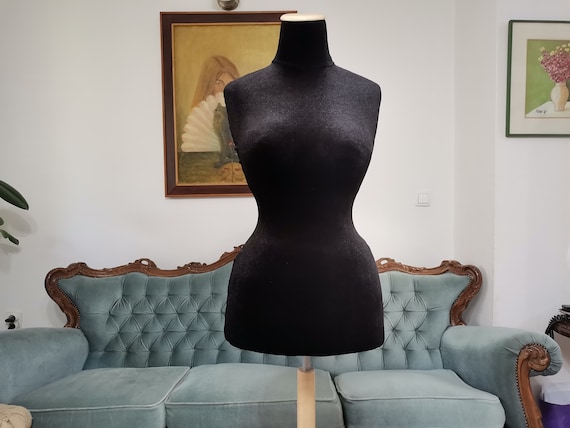This photograph captures a slightly cluttered, predominantly white room adorned with various decorative elements. Central to the image is a black dress form with an hourglass figure, mounted on a wooden stand. The dress form, headless and armless, prominently blocks part of an older painting on the white wall behind it. The visible portion of this painting appears to depict a young woman partially obscuring her face with a white fan. 

In the background, a large, ornate teal couch with dark wood trimming and intricate detailing is prominently featured. The couch's light blue velvety upholstery adds a touch of elegance to the scene. The left side of the photo partially captures the leaves of a plant, while the right side is cut off, showing just a glimpse of a second piece of artwork, likely a photograph or painting of a vase with flowers. 

On the floor, small objects such as plugs, cushions, and possibly more plants add to the room's slightly disorganized appearance, hinting that this could be either a home or a tastefully cluttered boutique with an antique flair.